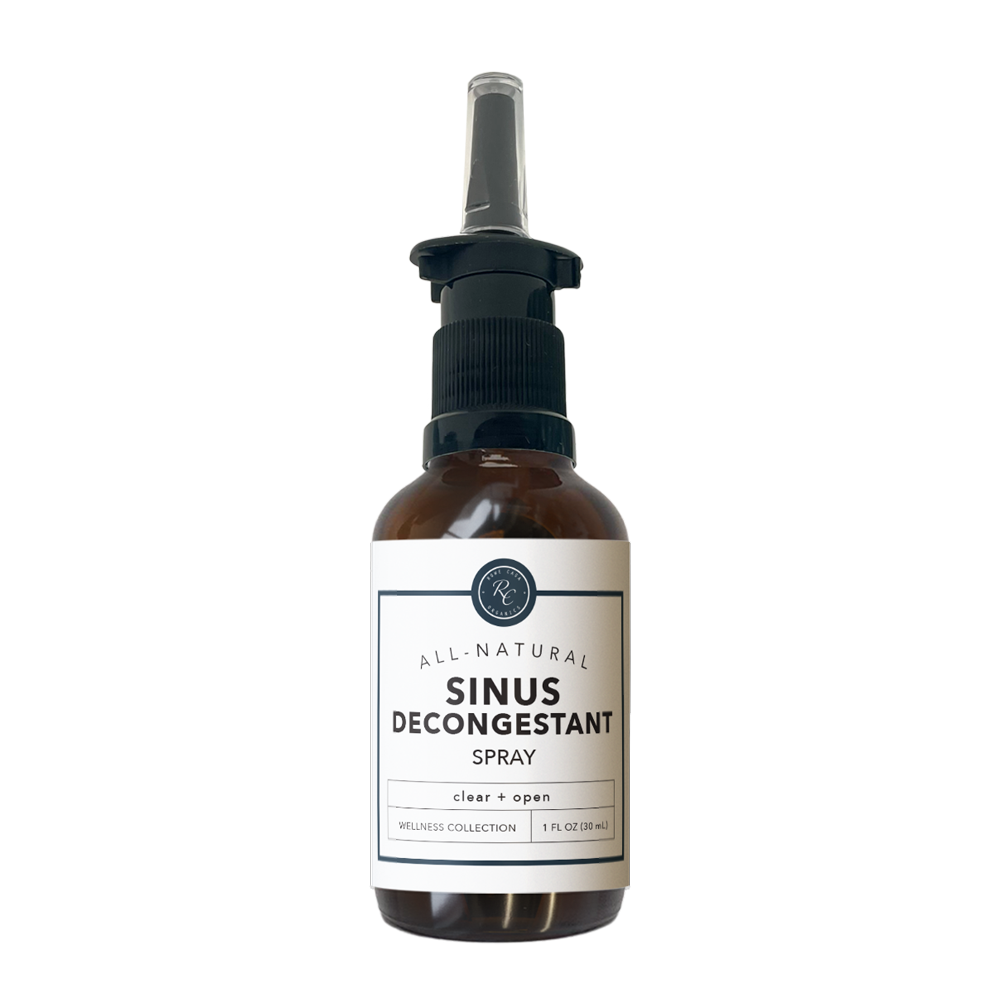The image showcases a single small spray bottle prominently centered against a white background. The bottle itself is transparent brown with a black spray nozzle, which includes a clear plastic cover. The label on the bottle features a white background with a green border and dark green text that reads "All-Natural Sinus Decongestant Spray." Below this, in smaller text, it states "Clear + Open." The product is part of the Wellness Collection and is indicated to be one fluid ounce (30 ml). The dark color of the bottle obscures the liquid inside, giving it a translucent yet opaque appearance.